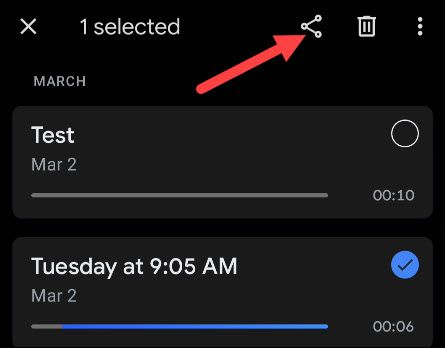Screenshot Description:

The screenshot features a black background with white and light gray text. At the top left corner, there is a header that reads "One Selected," accompanied by an "X" symbol. Next to this, there is a share icon depicted as three small circles connected by two lines. A large red arrow points towards this share icon for emphasis. In the upper right corner of the screenshot, there are a trash icon and an ellipsis (three small dots) in a row.

Below this header, the word "MARCH" is prominently displayed in all capital letters. Beneath "MARCH," there are two horizontally aligned rectangles with rounded corners stacked on top of each other.

- The first rectangle contains the text "Test, March 2."
- The second rectangle shows the text "Tuesday at 9:05 a.m., March 2," along with a blue circle containing a checkmark and a blue line below it.

This detailed layout provides a clear and organized view of the elements within the screenshot.